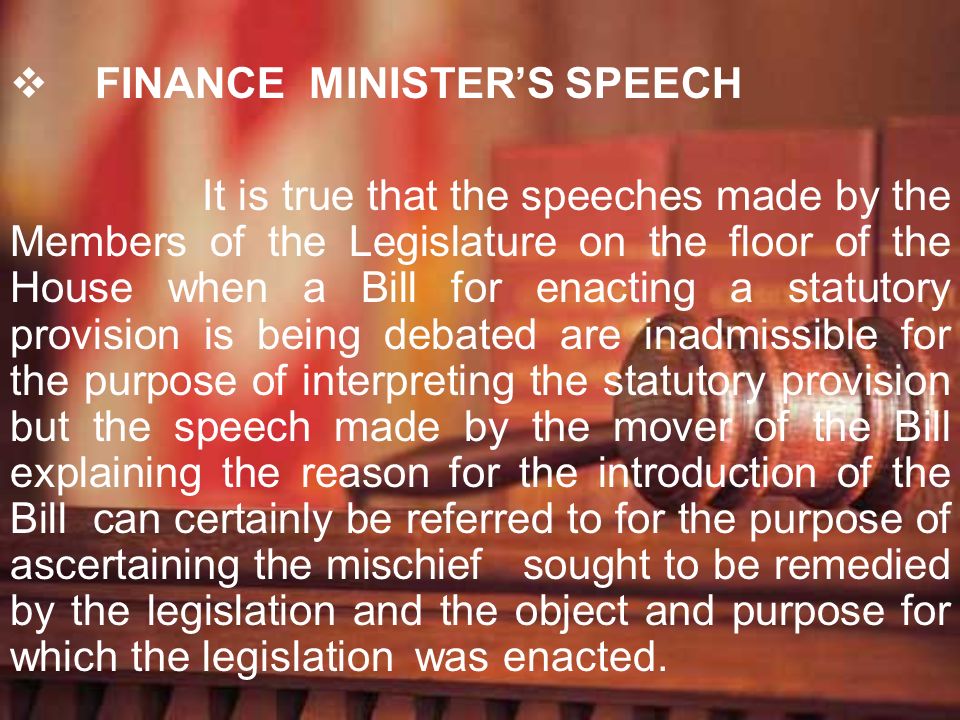The image depicts a PowerPoint presentation with a text-heavy slide. The background of the slide is slightly blurry but shows a judge's bench with a wooden gavel and some books, accompanied by a flag to the left of the chair. The image features overlayed white text. The heading at the top, in bold and capitalized white letters, reads "Finance Minister's Speech." Below this header, the slide contains a lengthy article in white text: "It is true that the speeches made by the members of the legislature on the floor of the House when a bill for enacting a statutory provision is being debated are inadmissible for the purpose of interpreting the statutory provision, but the speech made by the mover of the bill explaining the reason for the introduction of the bill can certainly be referred to for the purpose of ascertaining the mischief sought to be remedied by the legislation and the object and purpose for which the legislation was enacted." The background incorporates hues of red, brown, white, and a little bit of yellow.